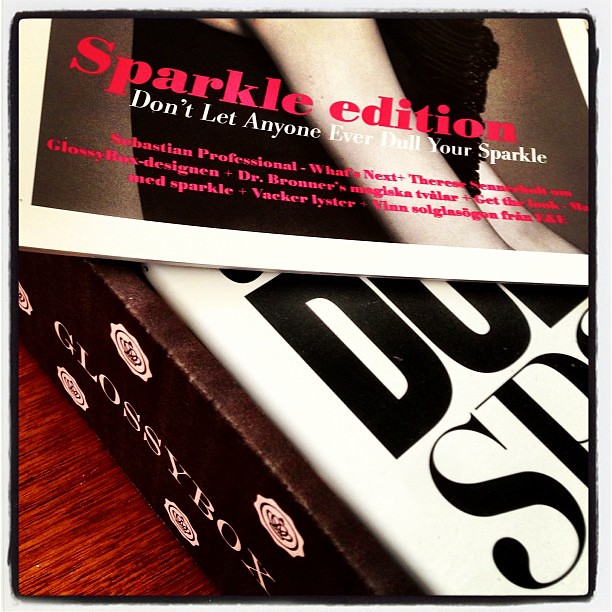A close-up, square photograph, possibly edited with Instagram filters for higher contrast, shows the bottom section of a magazine or a photograph placed on top of a gift box on a wooden table or desk. The visible part of the photograph features a woman’s arms and midsection, clad in a dark dress. Prominent pink text at the top of the photo reads, "Sparkle Edition," with white text underneath that advises, "Don't Let Anyone Ever Dull Your Sparkle." Below this, smaller red text includes phrases like "Sebastian Professional," and other partially readable lines. The white gift box beneath the image bears black lettering on its top and has the logo "Glossy Box" visible on its side.